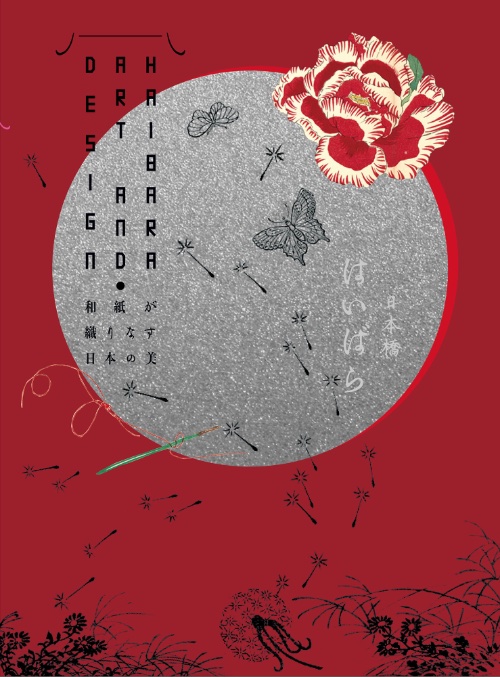This vertical rectangular image showcases a vibrant red background with a large grayish-white circle at its center. Adorning the circle are intricate designs, including a red flower with yellow bristles and delicate black butterflies. Gracefully entwined in the composition are green plants and additional small flowers. Towards the bottom, black splotches punctuate the red expanse, creating a contrast that leads the eye upward. Both side margins feature oriental characters in white—possibly Japanese or Chinese—adding an element of mystery to the art. On the upper left side, another set of unreadable oriental characters may explain more about the image. This poster, blending English phrases and Asian script, evokes the essence of Japanese art, weaving together text, floral motifs, and gentle arrows within a sophisticated, minimalist design.